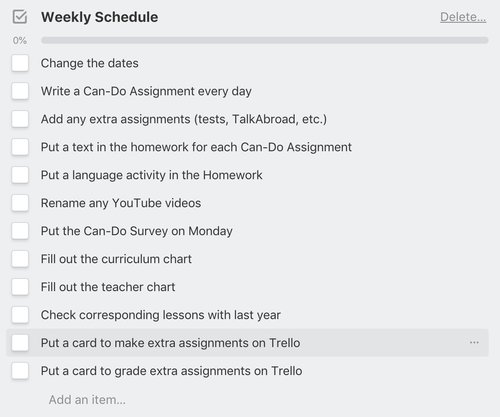The image depicts a "Weekly Schedule Checklist" with a light grey background. At the top, there is a grey square containing a tick mark, positioned next to the bold, black text that reads "Weekly Schedule". To the far right, there is an option to delete the checklist. Below the header, a progress indicator shows "0%" with an unfilled bar, suggesting that none of the listed tasks have been completed.

The checklist consists of several items, each accompanied by an empty white tick box. The tasks are listed in black text and include:

1. Change the dates
2. Write a can-do assignment every day
3. Add any extra assignments (e.g., tests, talk abroad, etc.)
4. Put a text in the homework for each can-do assignment
5. Put a language activity in the homework
6. Rename any YouTube videos
7. Put the can-do survey on Monday
8. Fill out the curriculum chart
9. Fill out the teacher chart
10. Check corresponding lessons with last year
11. Put a card to make extra assignments on Trello
12. Put a card to grade extra assignments on Trello

The task "Put a card to make extra assignments on Trello" is currently highlighted in a slightly darker grey shade, signifying it's the active selection. Beside this task, there are three vertical dots, indicating additional options or settings. Additionally, at the bottom of the checklist, there is an option to add another item.